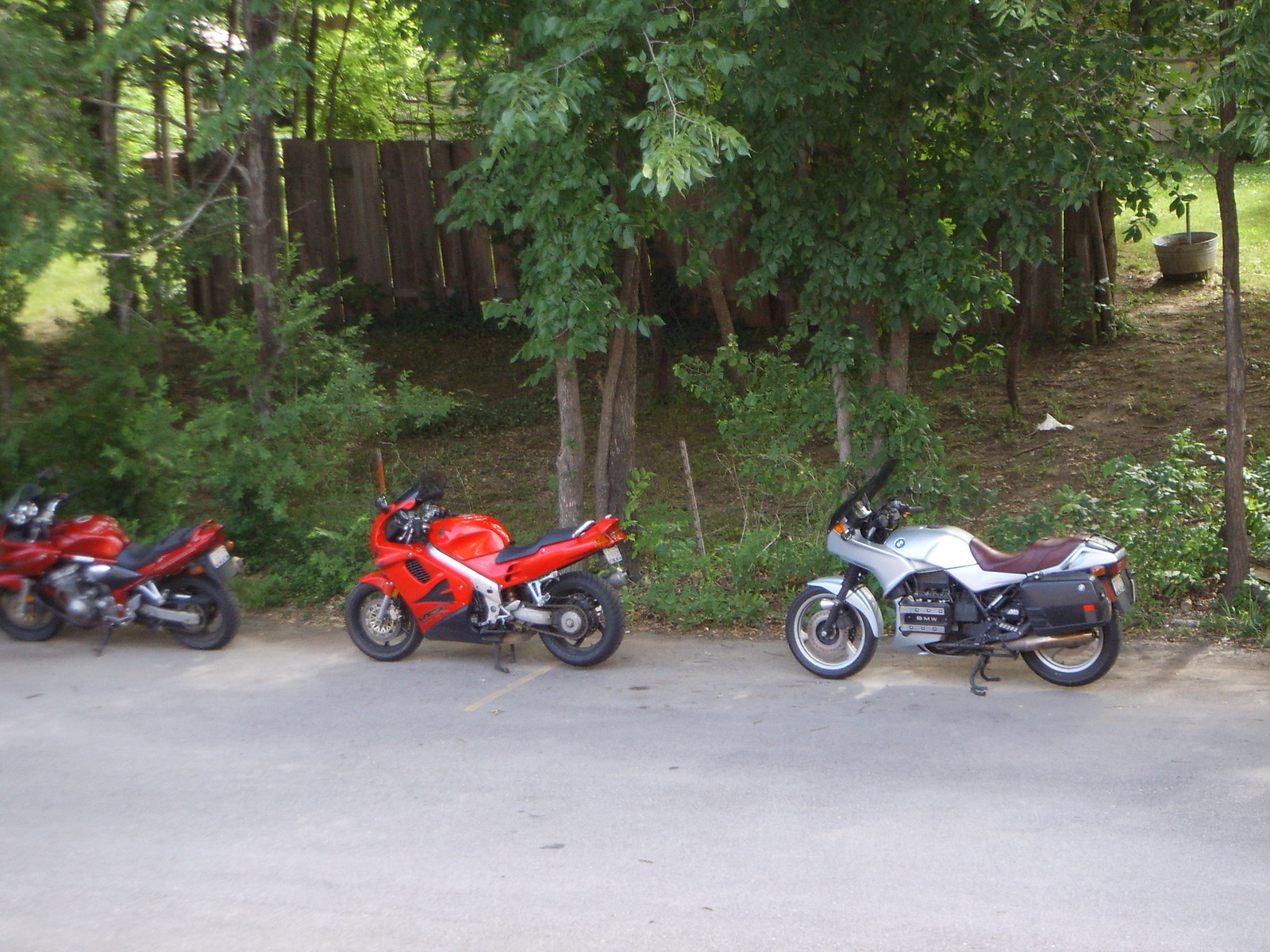This is a detailed color photograph capturing three distinct motorcycles parked on a light gray, somewhat whitish road that appears to have some sand and dirt on its surface. Each motorcycle is facing left, and from right to left, we have a silver motorcycle with a maroon seat and black trim, a bright cherry red motorcycle with black trim, and a dark apple red motorcycle with a black seat, with its left edge just cut out of the frame. The motorcycles are close to a brown wooden fence that runs through the middle of a hill, behind which a tall, brown, and thin stand of trees with abundant medium green leaves stretches skyward. Sunlight filters through these trees, illuminating bright green grass in the background. There are also some green plants and shrubs near the roadside area. In the upper right-hand corner of the photograph, a large silver drum or tub is visible near the trees. The photo captures a clear daytime scene, enhanced by the sunlight streaming through the foliage.